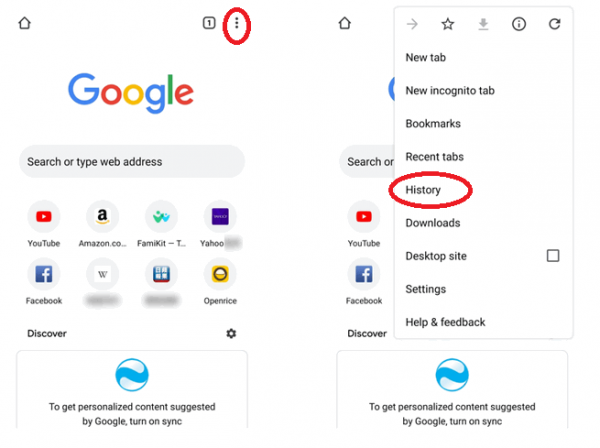This image, taken from a cell phone, showcases two screenshots side by side, with specific elements circled in red, likely as part of a tutorial on website usage. 

On the left screenshot, the browser is open to the Google homepage, characterized by its multicolored logo. In the top right corner, there is a numeral one encased in a square, adjacent to which are three vertical dots emblematic of a settings or options menu. These dots are encircled in an egg-shaped red outline. Below the Google logo, the prompt to "Search or type web address" is visible, accompanied by various icons including YouTube, Amazon, FamilyKit, Yahoo, and Facebook, with two additional icons blurred for privacy. The final icon in the visible row is labeled Opience. At the bottom of the screen, text suggests turning on sync to get personalized content via Google Discover.

The right screenshot displays a pop-up menu with different categories, and the term "History" is prominently circled in red, emphasizing its importance in the instructional context.